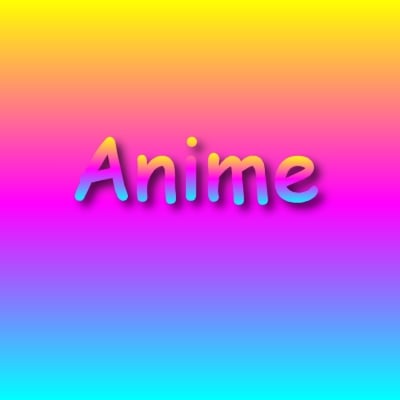This vibrant and colorful image prominently features the word "anime" in the center, designed in a rainbow color scheme. The background transitions smoothly from yellow at the top, through shades of orange, pink, purple, and dark purple, finally ending with blue and light blue at the bottom. The letters "anime" are also filled with the same gradient, starting with yellow at the top and transitioning through the same colors to blue at the bottom of each letter. The text is centrally placed, with ample space on either side, making the overall composition appear balanced. The entire image gives the impression of a creatively designed poster, suitable for various settings such as an art gallery, a home decor piece, or a vibrant page in a coloring book.